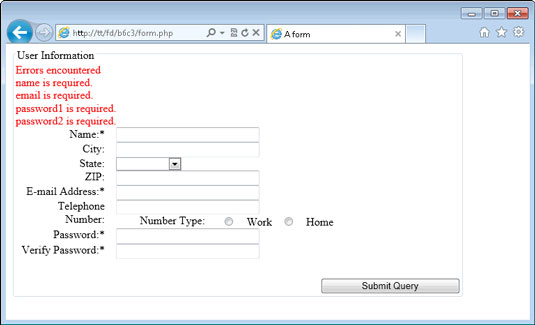This image is a screenshot of a computer screen showcasing a web form interface. In the top left corner, there is a blue circle with a white back arrow, and to its right, a smaller circle with a forward arrow. The top right corner features standard window control buttons: an "X" to close the screen, a square to maximize it, and a minimize button. Beneath these controls are a home button, a star button, and a settings button.

Right next to the back and forward arrows, there is a search bar containing a web address, followed by another bar labeled "aform," which includes a close (X) button on the far right. This section appears to be part of a web browser interface with potentially another tab open.

The body of the image displays text and input fields for a user form. In the top left corner of this section, the text "User Information" is written in black. Below it, in red, is "Errors Encountered" accompanied by error messages: "Name is required, Email is required, Password 1 is required, Password 2 is required."

The form fields are listed directly underneath and slightly to the right, in the following order from top to bottom: Name, City, State (with a dropdown menu), Zip, Email Address, Telephone Number, Password, and Verify Password. Each field has corresponding text boxes except for "State," which features a dropdown menu. Between the "Telephone Number" and "Password" fields, there are two radio buttons to select either "Work" or "Home."

In the bottom right corner, there is a "Submit Query" button to finalize the form submission.